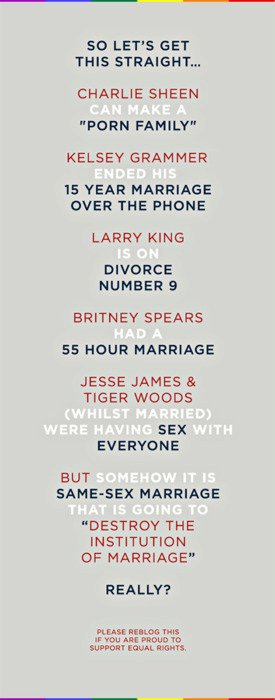The image is a tall rectangular promotional flyer with a dark gray background and thin rainbow-colored borders at the top and bottom. These borders consist of small segments of purple, blue, green, yellow, orange, and red. The central text is arranged into several lines with varying colors and fonts.

The main text begins with, "SO LET'S GET THIS STRAIGHT…" in bold blue capital letters on the first line. Below it, in alternating red, white, and blue letters, it states:

- "Charlie Sheen can make a "porn family"."
- "Kelsey Grammer ended his 15-year marriage over the phone."
- "Larry King is on divorce number nine."
- "Britney Spears had a 55-hour marriage."
- "Jesse James and Tiger Woods, whilst married, were having sex with everyone."

Following these points, the flyer challenges the reader by saying, "But somehow it is same-sex marriage that is going to 'destroy the institution of marriage'." in red letters, ending with, "REALLY?" in white text.

The message concludes with a plea in white text: "Please reblog this if you’re proud to support equal rights."

The image juxtaposes examples of heterosexual relationships' failures and infidelities to question the criticism of same-sex marriage, supporting equal rights for all.